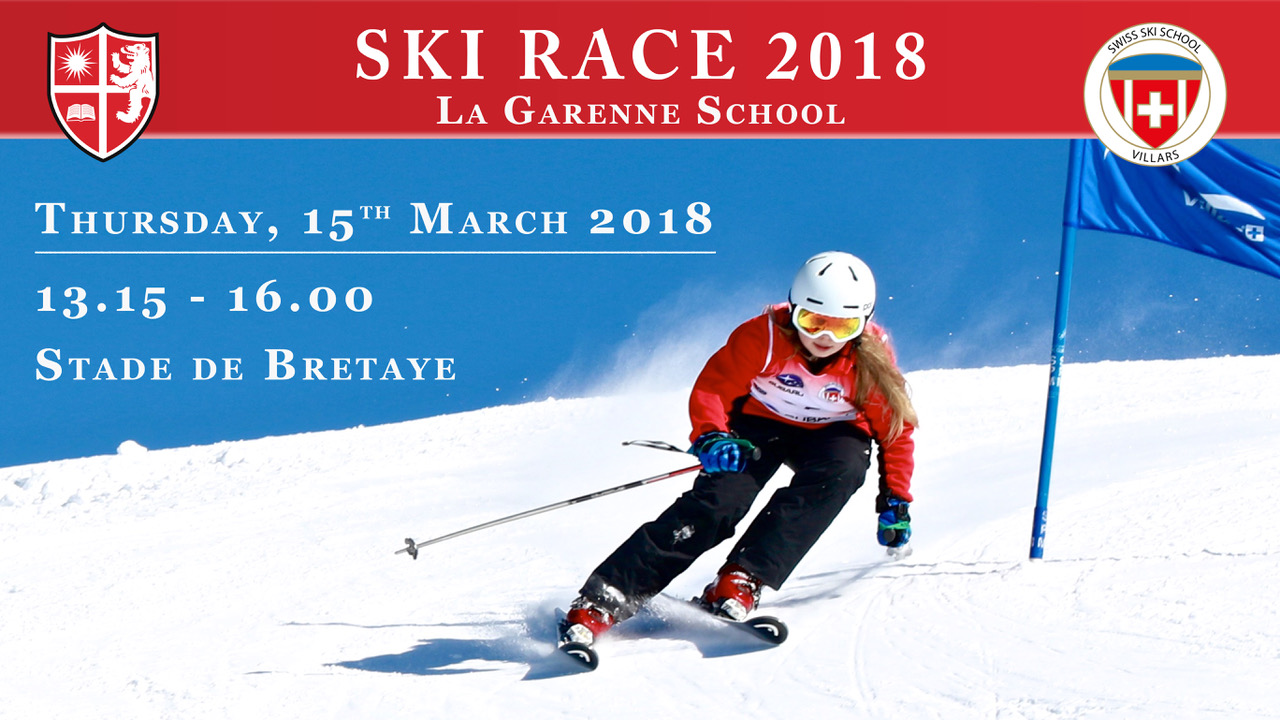This detailed advertisement for Ski Race 2018 features a vibrant and dynamic layout. At the top, a striking red horizontal banner spans the width of the poster. On the left side of this banner, a detailed heraldic shield is depicted in red, white, and black, featuring a lion, a sun, and a book. To the right, a white circle contains the Swiss shield with a red background and white cross, accompanied by the text "Swiss Ski School" above and "Villars" below. The bold white lettering in the center of the red banner reads “Ski Race 2018,” with "Le Garon School" written directly below in a smaller font.

Dominating the center of the poster, a clear blue sky frames the scene, which includes a crisp snowy landscape beneath. A female skier, in full winter gear, takes the spotlight. She is captured skiing downhill in a red ski jacket, black pants, blue gloves, red boots, white helmet, and ski goggles. She elegantly maneuvers past a blue flag, positioned to her right, marking her path as she makes her descent on the snowy slope.

Additional details are presented in white text to the left of the skier, set against the serene blue sky: “Thursday, 15th March 2018, 13.15 to 16.00,” followed by the location, “Stade de Bretaye.” This visually engaging and informative advertisement captivates viewers, drawing them into the excitement of the upcoming ski race event.